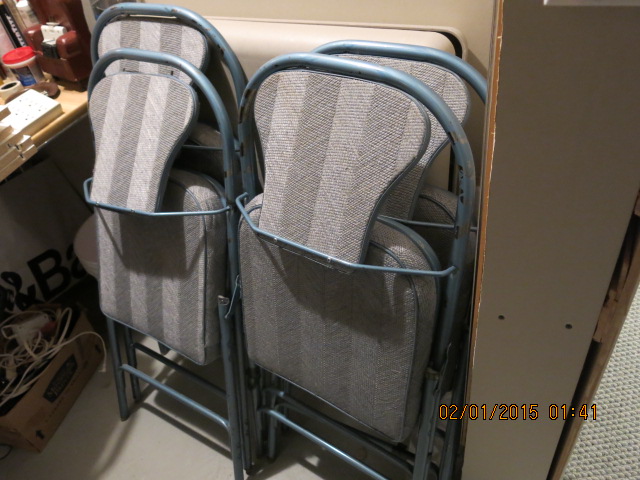The image likely depicts a backstage area of a theater or movie set, captured on February 1, 2015, at 01:01. In the center of the image, four foldable chairs with blue frames and grey cushioned seats and backs are leaned against each other along a wall. The chair frames show signs of wear, revealing some silver underneath the peeling blue paint. To the left of the chairs is a desk cluttered with indistinguishable items, including makeup products and a small white container with a blue label and red cap. Beneath the desk lies a brown cardboard box filled with charger cables and other miscellaneous wires. Behind this desk, there's a large, partially visible box marked with the letter "B." On the right side of the image, a door is hinged open, allowing a glimpse of the grey-carpeted floor. The overall scene is one of organized chaos, typical of behind-the-scenes environments.